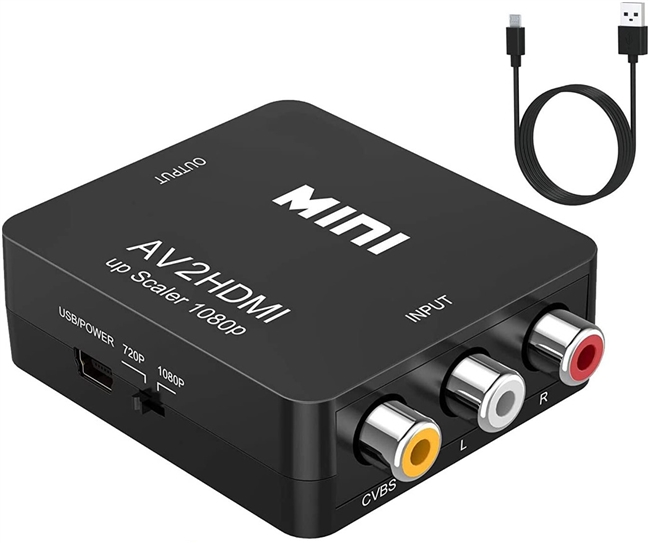This image features a close-up shot of a black plastic HDMI upscaler box, designed for converting AV inputs to HDMI output. The device prominently displays the text "Mini AV to HDMI Upscaler 1080p" at the top. On the right-hand side, three distinct input ports in yellow, white, and red are arranged vertically; these are labeled "CBVS," "L," and "R," respectively, indicating connections for composite video and stereo audio. To the left, there's a USB power port accompanied by a switch that toggles the output resolution between 720p and 1080p. In the top right corner of the image, a coiled charger with a long cord is visible, featuring a USB connector on one end and a probable USB-C connector on the other.